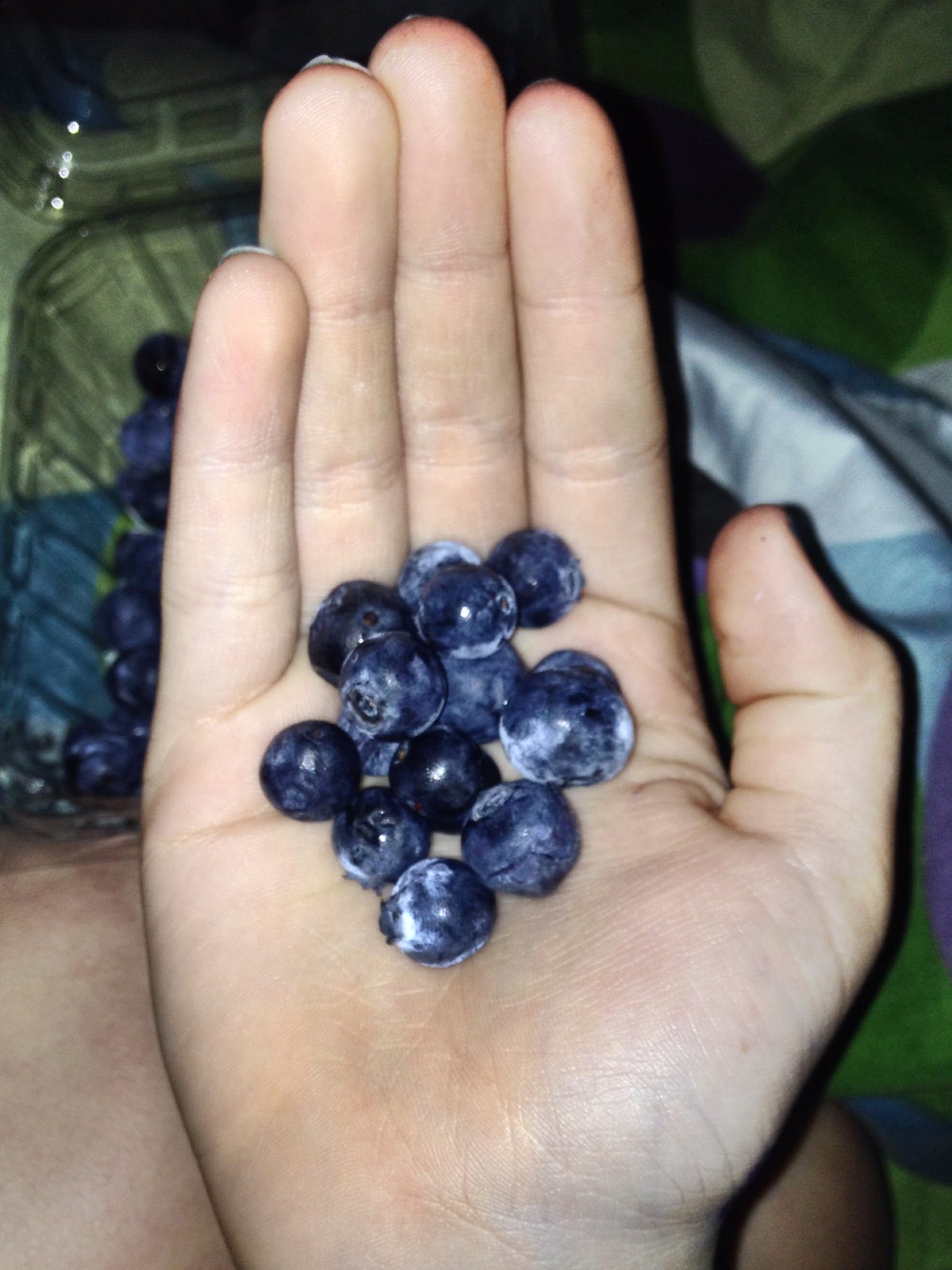In this photograph, a person's right hand, palm up and flat, is prominently displayed, holding a small pile of about 14 blueberries. The blueberries are of varying sizes and shades, ranging from dark blue to lighter hues with characteristic little white coatings that often wash off under water. The person's hand, featuring short nails and belonging to a Caucasian individual, occupies the majority of the image, with their knees visible at the bottom left.

The background reveals several additional details. Behind the hand, there is a clear plastic package containing more blueberries, with the lid partially visible in the upper left corner of the image. To the right of the hand, a fabric in shades of green, purple, light blue, and dark blue adds texture and depth to the scene. Below the hand, the person's skin, likely their legs, can be seen. The photograph is dramatically lit, with a harsh light source illuminating the hand and casting deep black shadows in the top right area, enhancing the contrast within the image.